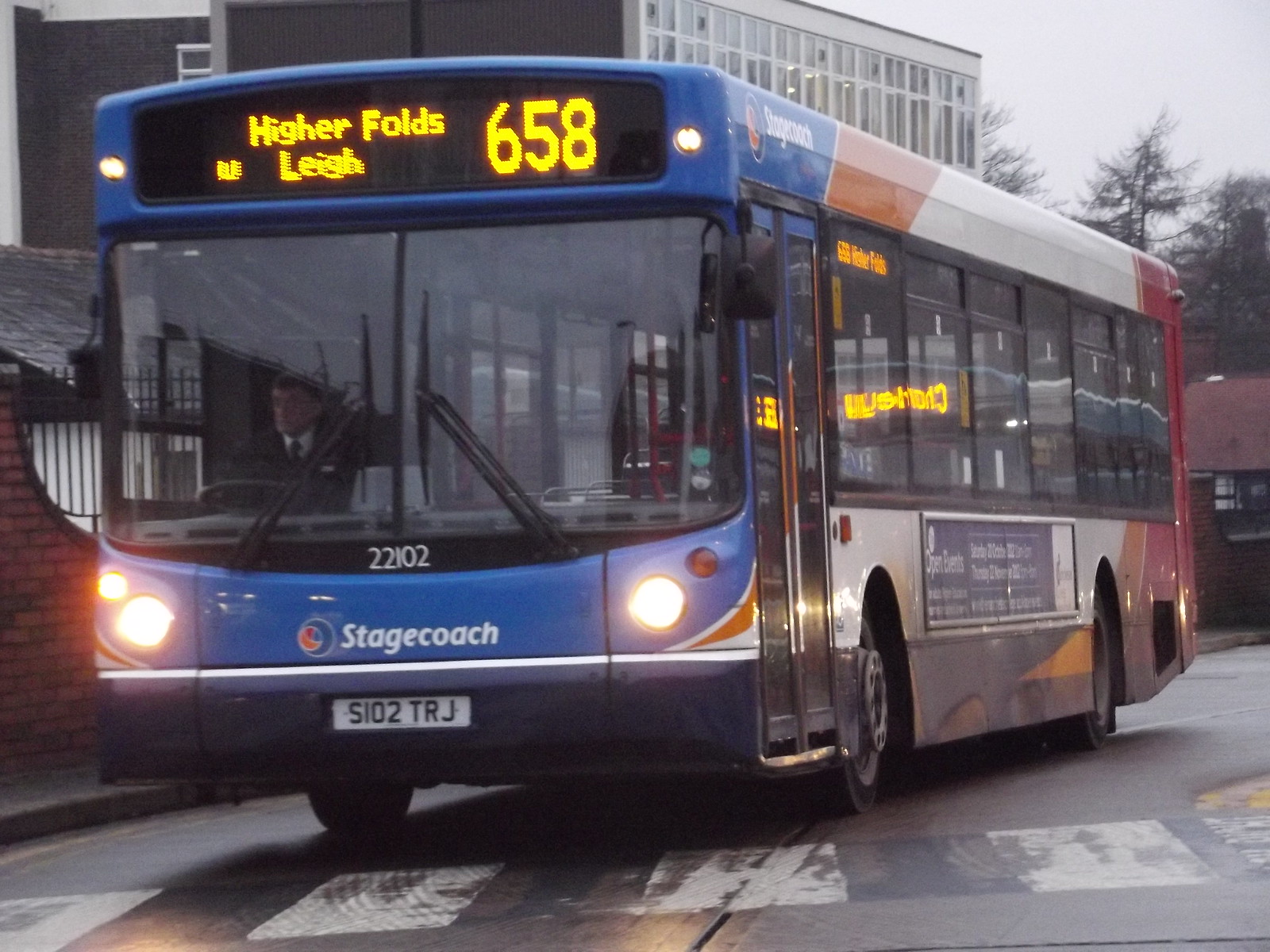This image captures a blue city transit bus with red and white stripes that's currently moving. The bus is facing the camera but angled slightly to the left, highlighting its front, which displays the word "Stagecoach" along with the company logo – a circle with blue, orange, and red colors. The license plate reads S102 TRJ. Positioned over a crosswalk with thick white painted areas, the bus is illuminated by its headlights, suggesting a gray day. The bus displays its route and destination, "Higher Folds Lee 658," in yellow digital lettering at the top. The driver is on the right side of the bus, indicating it might be in England. Adjacent to the bus on the left is a sidewalk against a red brick wall. The background features a tall office building with many windows. An advertisement in blue and white can be seen at the bottom of the bus, underneath the windows.